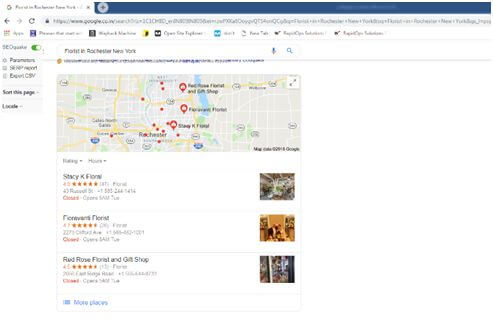Screenshot depicting a search for florists in Rochester, New York on what appears to be Microsoft Edge. Despite the low image quality, it's clear that the results highlight several florists, including Stacy K. Floral and Red Rose Florist and Gift Shop, both of which boast high ratings of 4.9 stars. The search results display a segment of a map of Rochester, marked with various red location icons indicating the florists' positions. Each florist listing includes a name, rating, and a small accompanying photo, though the photos are too pixelated to discern any specific details. The background of the screenshot is predominantly white, providing contrast to the text and map elements.